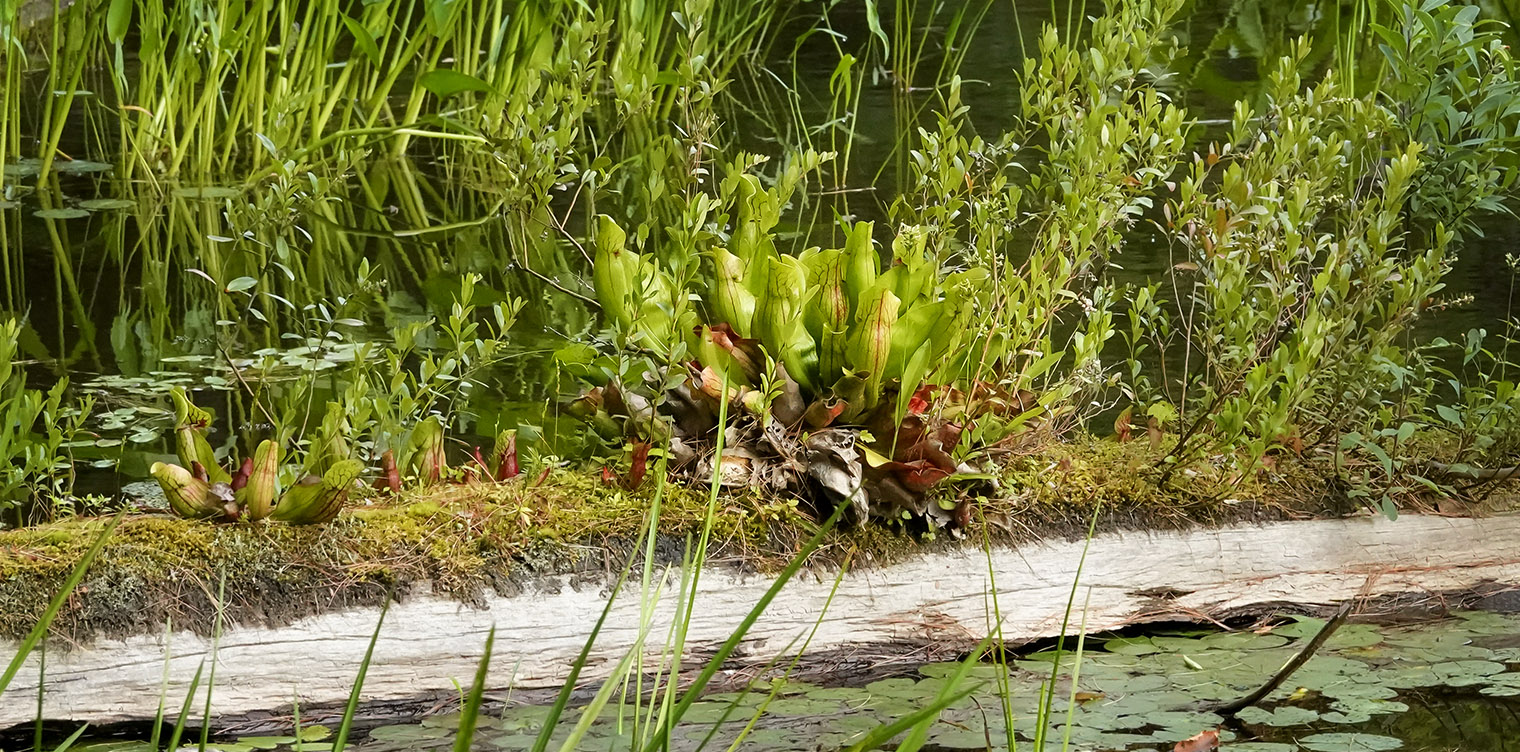This photograph captures a lush, vibrant wetland scene, possibly at the edge of a pond or within a swamp. Dominating the image is a rich array of green vegetation, including a variety of pitcher plants with their distinctive insectivorous features, moss, and bog plants. Among the greenery, cattails rise prominently in the background, adding height to the dense tapestry of plants. In the foreground, lily pads float serenely on the water’s surface, reinforcing the wetland setting. A log or linear stump stretches across the scene, providing a substrate for some of the plants. This log could be part of the pond's bank or simply a fallen tree now teeming with life. The dense cluster of plants is punctuated with patches of red and brown, particularly seen on the lower parts of the pitcher plants and some leaves, adding a striking contrast to the predominantly green landscape. The photograph, taken in daylight, shows textures and colors with great clarity, reflecting the rich biodiversity and intricate ecosystem of the wetland.